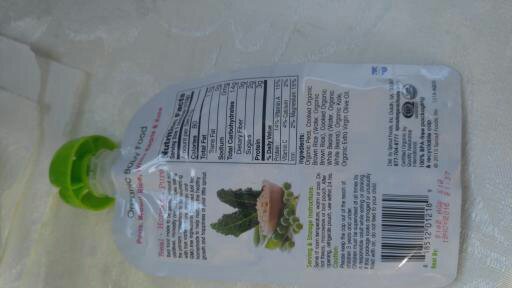In this image, the backside of a package of baby food is displayed, tilted on its side, suggesting the photograph was taken horizontally. The package itself is white and features a green, squeezable cap. The image focuses on the nutrition information panel, though the text is largely illegible due to the small size and poor focus of the photograph. "Organic Baby Food" is discernible at the top in larger font, highlighting the product's organic nature. However, the rest of the details, including the list of ingredients and specific nutritional information, are blurry and difficult to read.